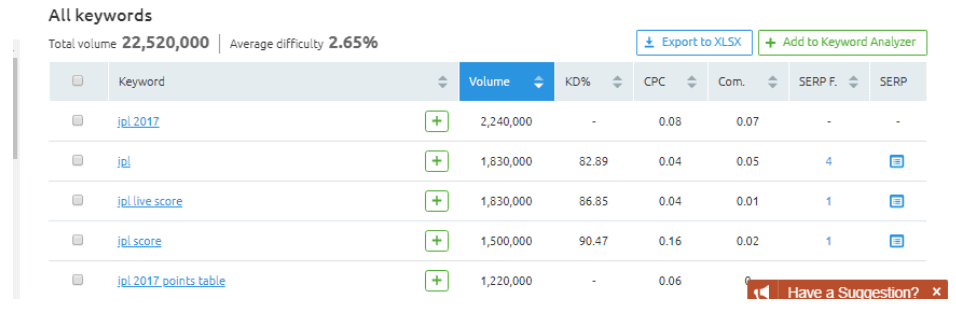The image displays a user interface of a keyword analysis tool. At the top, the header is prominently titled "All Keywords" in bold, black text. Below this, key metrics are summarized: "Total Volume: 22,520" and "Average Difficulty: 2.65%". 

To the right of these summaries, there are options labeled "Export" and "Add Keyword Analyzer." 

The interface is divided into several columns:
1. **Checkboxes:** The first column contains checkboxes for selecting individual keywords.
2. **Keyword:** The next column lists various keywords.
3. **JPJ Scores 2017:** This column presents scores from 2017 related to JPJ, with a detailed list of scores.
4. **Add (+):** An option to add more keywords is available here.
5. **Volume:** This column shows the search volume for each keyword, with numbers ranging from 1 million to 2 million.
6. **KD%:** Indicates the keyword difficulty percentage.
7. **CPC:** Lists the cost-per-click for each keyword.
8. **COM:** Abbreviation details not specified, it could be 'Competition' or another metric.
9. **SERP:** Search Engine Results Pages data, split into columns "F" and "SERP" for further specifics.

Some columns also have dropdown menus that allow users to modify the displayed data.